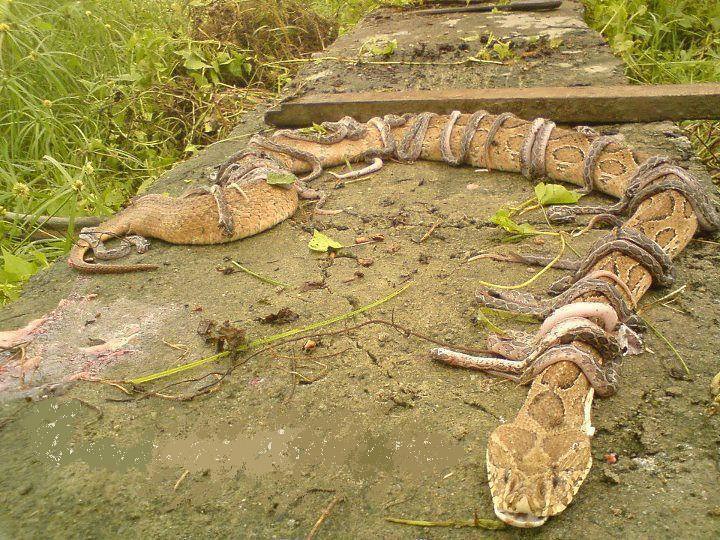The photograph showcases a large brown and tan python, detailed with darker brown spots and gold speckles, laying on a muddy, greenish surface that seems to be part of a path or enclosure. The python's head, located in the lower right corner, lies flat with its mouth open, revealing a white bottom jaw and gray eyes staring towards the camera. Scattered across the python's body are numerous smaller snakes, appearing lifeless, with some draped over the larger snake and others lying with their soft white bellies exposed. The ground is textured with muddy soil, and in the top left corner, long, unkempt green grass can be seen. In the background, a dirty wooden plank extends off to the right, reinforcing the sense of a disordered or natural setting. Yellow flowers add a touch of color among the grassy surroundings, indicating it might have been taken on a sunny day. The scene is both fascinating and unsettling, emphasizing the eerie calmness and the possible lifelessness of the snakes present.